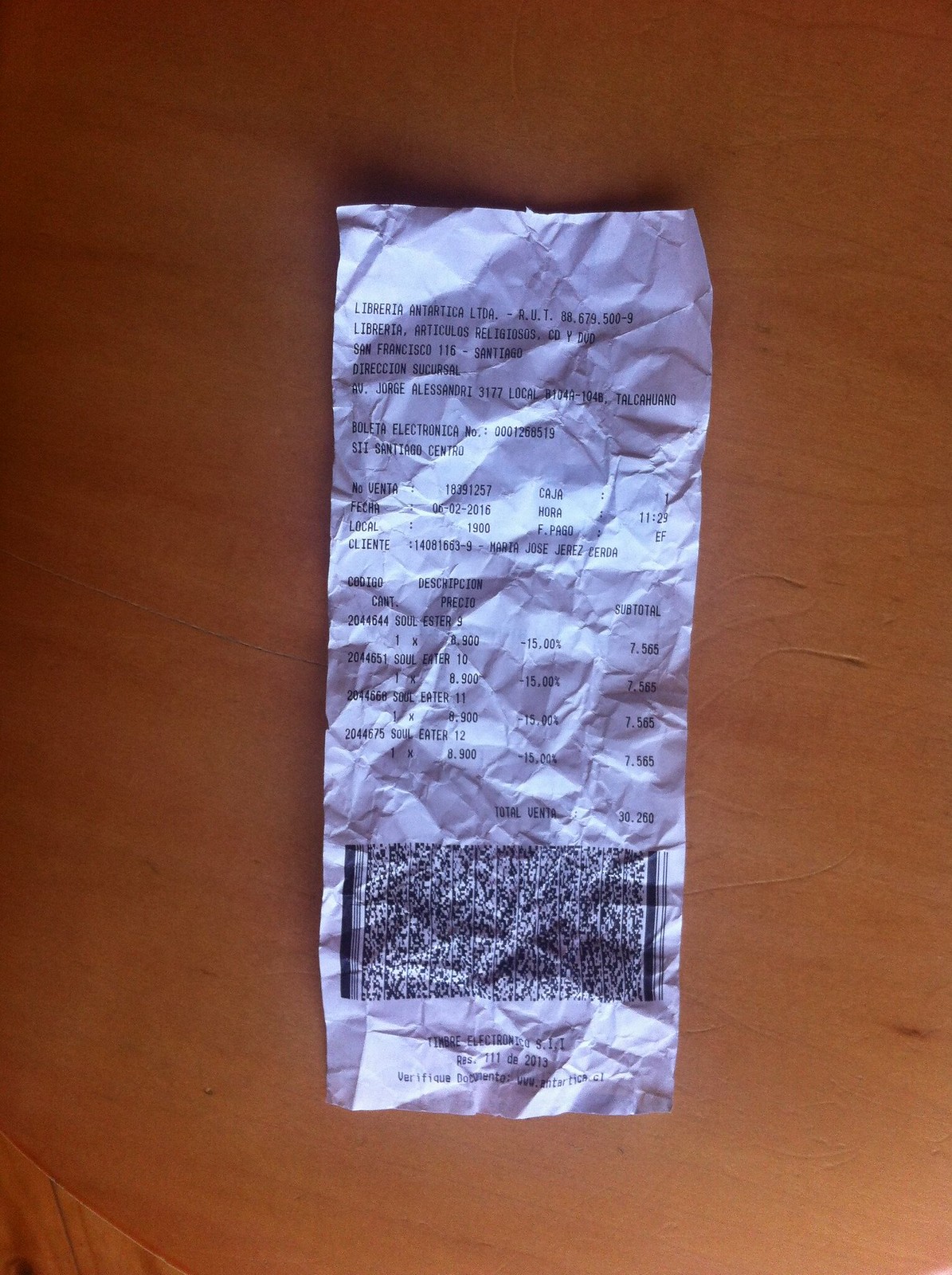A detailed top-down photograph captures a heavily wrinkled white receipt lying on a worn wooden surface, showcasing the receipt's many creases and crumples that cast various shadows and light areas. At the top of the receipt, printed in black text, is the header "Liberia Antarctica LTDA," followed by numbers such as "8.67 9.500 - 9" that are partially readable. Beneath this header, more black text is printed, including "San Francisco 115-10 San Santiago" indicating a possible address or location. 

Further down, the text becomes challenging to decipher due to language barriers, likely Spanish, as evidenced by phrases like "boleta electronica." Other numbers such as "00072" are also visible, contributing to the receipt's intricacy. 

The middle section lists various purchased items, although specific details are obscured by the receipt's condition. The bottom part of the receipt features a prominent barcode, accompanied by additional text that remains partially obscured or unreadable. The wooden surface below the receipt shows signs of wear, adorned with scratches and dents, adding to the photo's authentic, lived-in feel.